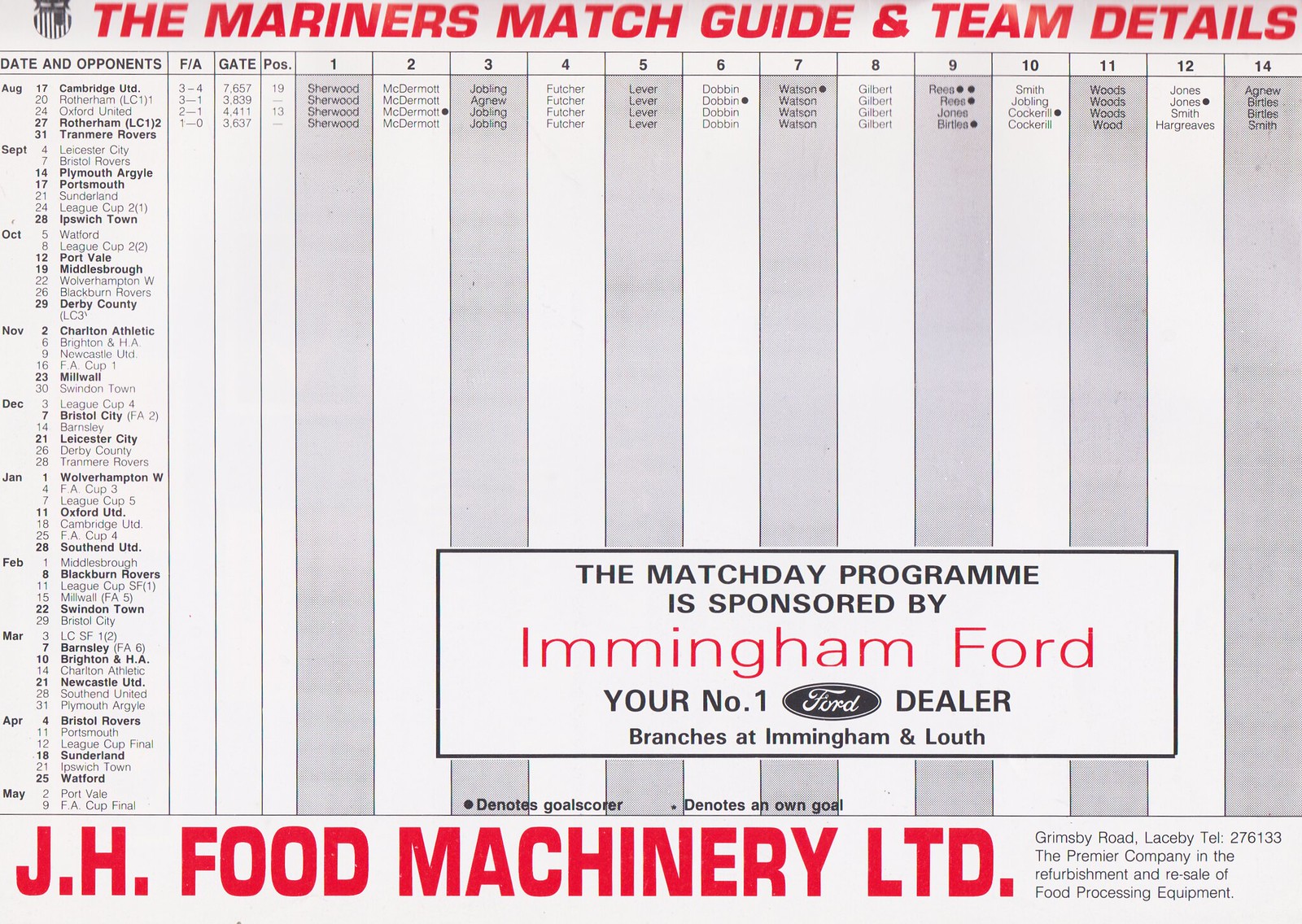The document is a detailed match guide and team details chart for a sports game. The title, "Mariners Match Guide and Team Details," is prominently displayed at the top in large red font. The left-hand side of the document is organized vertically with dates listed from August through May, and it specifies the teams and towns where the games will be held. The chart includes columns for additional information such as gate positions numbered from 1 to 14, match dates, opponents, and possibly some FA statistics. Midway, there's a rectangular advertisement box stating that the "Match day program is sponsored by Immingham Ford, your number one Ford dealer, with branches in Immingham and Louth." At the very bottom, also in bold red lettering, it reads "J.H. Food Machinery, Ltd., Grimsby Road, Laceby, telephone number 276133," which is noted as the premier company in the refurbishment and resale of food processing equipment.